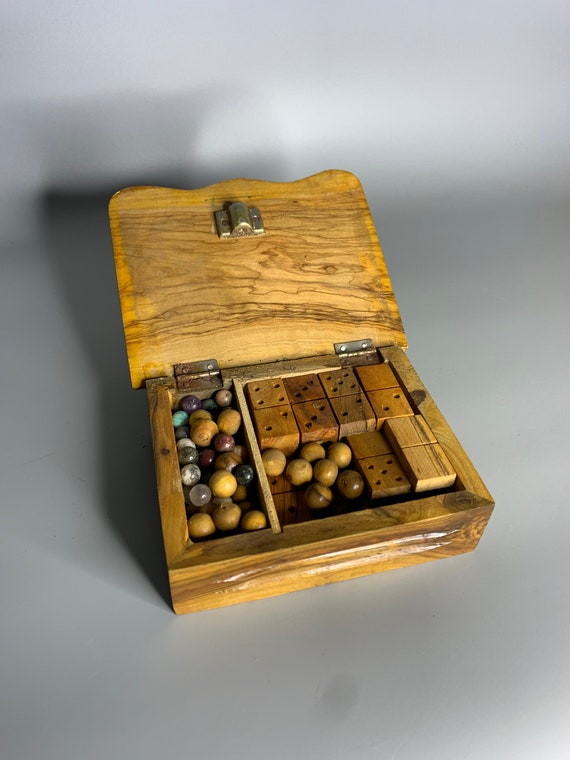This photograph showcases a small, old wooden box, approximately 5 inches in length, 4 inches in width, and 1.5 inches in height, placed on a light grey surface that fills the background. The light tan box, featuring brown streaks, is open, revealing its contents. The box is equipped with two metal hinges at the back and a clasp at the front. Inside, the box is divided into two sections. The left, smaller section contains an assortment of marbles, both wooden and glass, with some glass marbles in shades of blue, clear, and purple. The right, larger section holds wooden cubes, some of which are crafted like dice with drilled-out number holes, alongside additional wooden marbles. The box’s shadow is visible on the background surface, enhancing the depth and detail of the image.